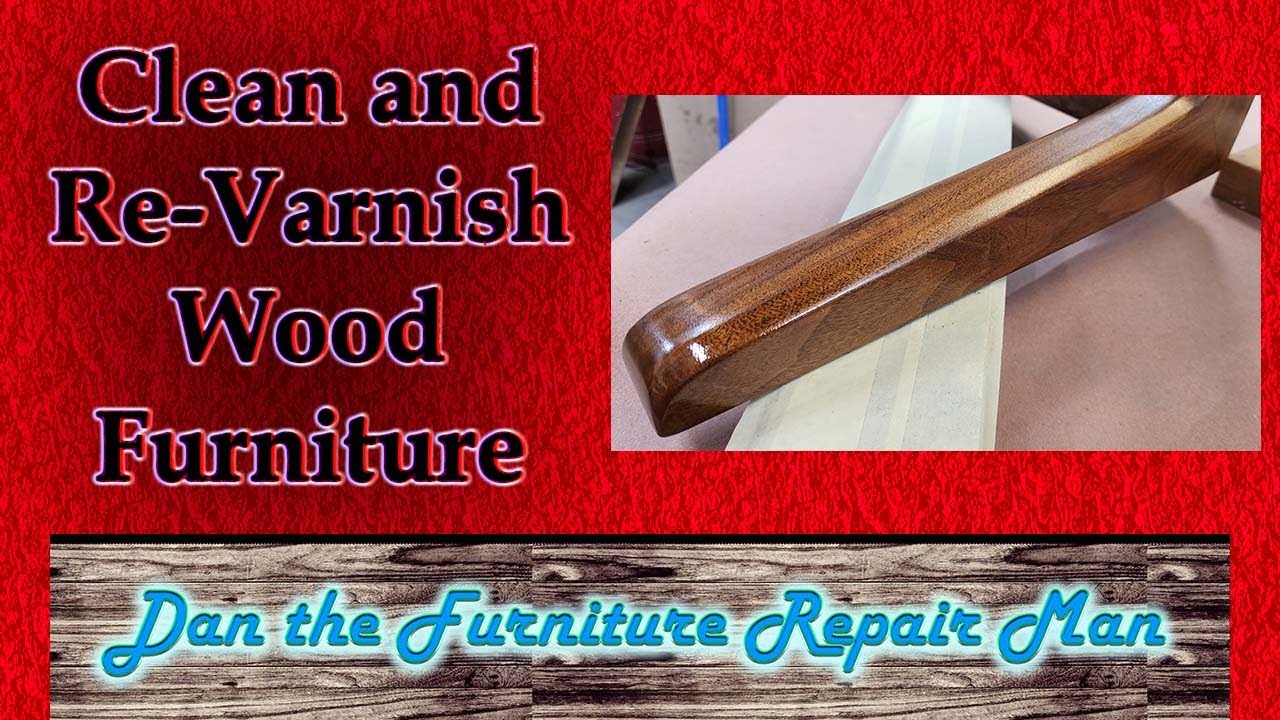The image features an amateurish advertisement for Dan the Furniture Repairman. The backdrop is a striking red, reminiscent of a basic PowerPoint slide template. Prominently displayed is text that reads "Clean and Re-varnish Wood Furniture." To the right of this text, there is a highly polished and shiny piece of wood, possibly part of a chair or another piece of furniture, showcasing Dan's expertise in wood finishing and sealing. At the bottom, the advertisement includes Dan's name in a memorable blue script font written over a piece of 2x4 wood that emphasizes the wood grain. Although the design lacks sophistication and cohesion, with mismatched textures and fonts, it still manages to communicate Dan's services effectively.